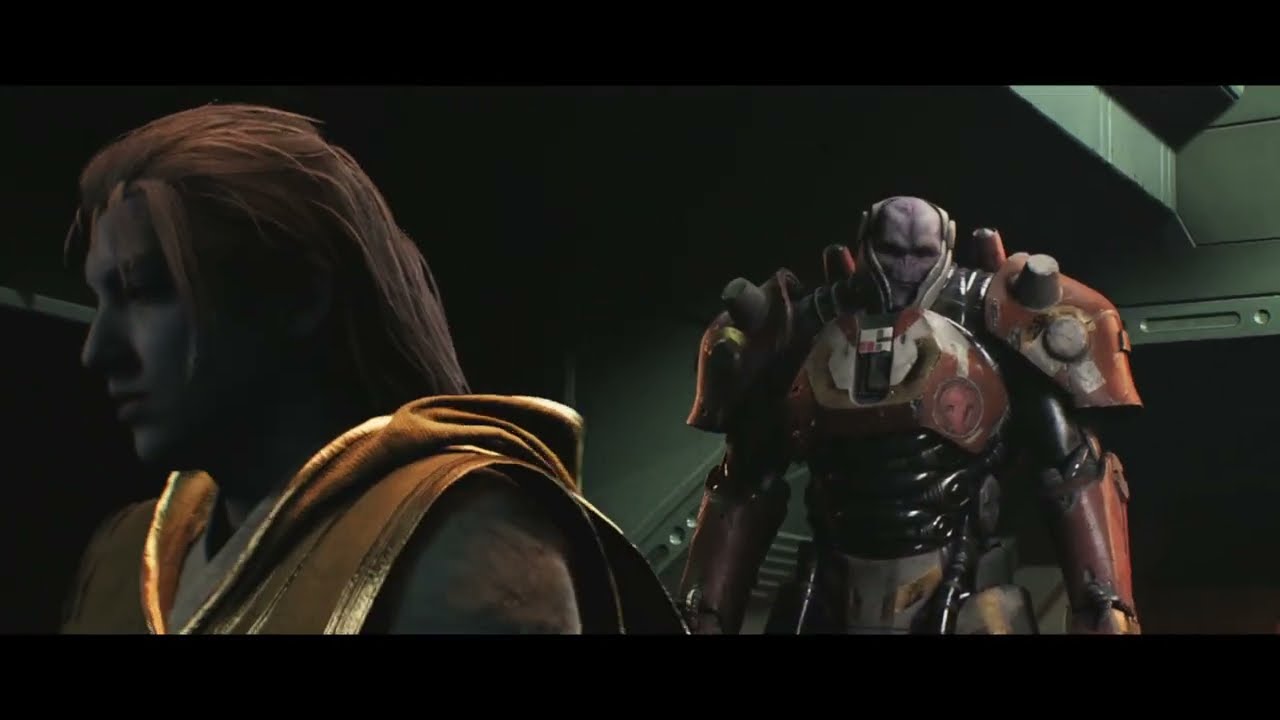The image appears to be a scene from an animated movie or video game, set inside a space station or spaceship. The scene is framed by thin black lines at the top and bottom. In the foreground, on the left side, there's a character with long, straight reddish-brown hair, gray skin, and wearing a sleeveless gold tunic-type shirt with a hood, along with a brown undershirt. This character's gender isn't immediately clear.

Behind this character, on the right side, stands an imposing figure that appears to be an alien or robot with humanoid features, clad in a large robotic armor. This character has a small, bald, gray head with pronounced eyebrows, no nose, just small nostrils, and a slit for a mouth. The armor is predominantly red with a black stomach area and purple face, with details like bolts or cup-like structures on the shoulders.

The backdrop includes gray walls and darker areas such as a shadowed doorway and corners, suggesting a dim, enclosed environment. The setting, rich with colors like gold, brown, grayish-blue, auburn, red, silver, light purple, and green, reinforces the high-tech, otherworldly atmosphere of the scene. The overall environment and character design hint that this is part of a larger narrative within a space-themed video game or movie.